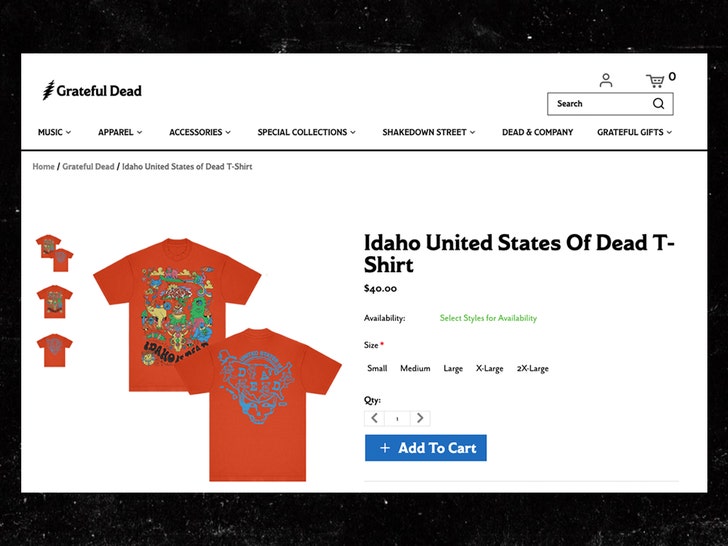A detailed website screenshot captures the Grateful Dead online store interface. In the top left corner, "Grateful Dead" is prominently displayed with a lightning bolt logo next to the word "Grateful." Directly beneath, a navigation menu provides links to various sections: Music, Apparel, Accessories, Special Collections, Shakedown Street, Dead and Company, Grateful Gifts. Adjacent to these links are a search bar, a user account icon, and a shopping cart icon.

The breadcrumb trail indicates the following path: Home / Grateful Dead / Idaho United States of Dead T-Shirt. Below this, an image showcases a red t-shirt with a psychedelic pattern on the front. A second image reveals the back of the same shirt, featuring the iconic Grateful Dead skull logo with the word "Dead" inscribed on it.

To the right, the text "Idaho United States of Dead T-Shirt" is displayed along with the price, $40. The availability section advises to "select styles for availability," listing sizes ranging from Small to 2X Large. The quantity is set to one by default, and a blue rectangle button labeled "Add to Cart" is ready for the user to make a purchase.

The entire screenshot is framed with a thick black border. The image is devoid of any people or animals and is focused solely on the website's vibrant, color-rich design.